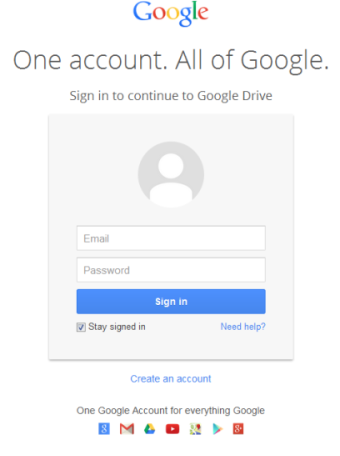The image depicts the screen of a smartphone displaying the Google Gmail sign-in page. The background is primarily white. At the top of the screen, the Google logo is prominently featured with the letters in their characteristic colors (blue, red, yellow, and green). Below the logo, grey text reads "One account. All of Google," followed by smaller grey text that says "Sign in to continue to Google Drive."

Further down, there's a grey section displaying a darker grey circular icon with the outline of a person, representing a user profile. Beneath this icon are two text boxes for user input: the first for the email address and the second for the password. Below the text boxes, a blue button with white text instructs the user to "Sign in."

Below the sign-in button, a small checkbox is marked, indicating "Stay signed in." To the right of this checkbox, blue text asks "Need help?" with a question mark.

At the bottom of the screen, the text prompts users to "Create an account," followed by a statement in dark grey or black font: "One Google Account for everything Google." The image also includes links to other Google applications such as YouTube, Google Drive, Gmail, etc.